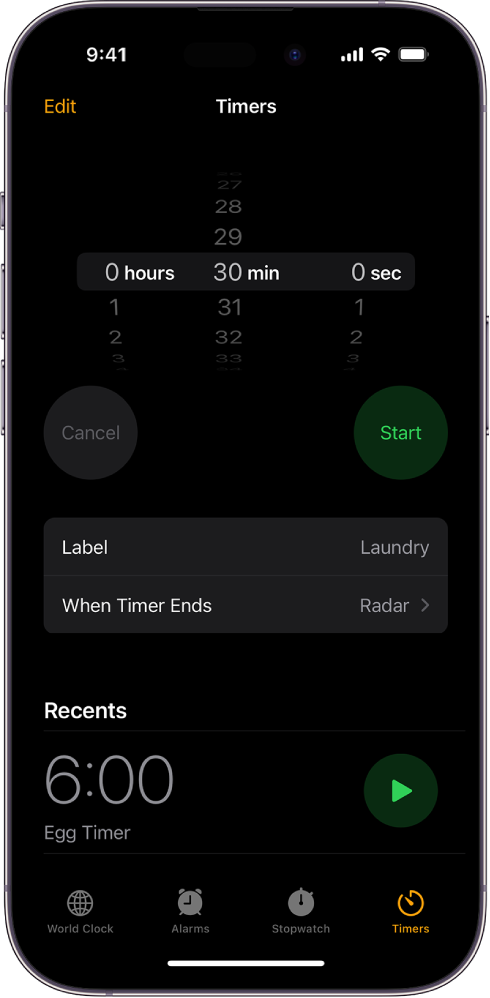### Descriptive Caption:

The screenshot captures the timer feature on an iPhone against a black screen. In the upper left corner, there's an orange "Edit" button, clearly indicating it is clickable. At the top center of the screen, "Timers" is displayed in white. Below this, there is a scrollable wheel where different times can be set. The timer is currently set to 0 hours and 30 minutes, which is highlighted.

In the upper right corner, the current time is shown as 9:41. Central to the interface, there's a prominent green oval "Start" button. Situated below this button is an area for setting labels, currently labeled as "Laundry." Beneath this, "When Timer Ends" is displayed in white, followed by "Radar," which allows you to set the type of alarm sound. 

Further down, there’s a "Recents" section in white, listing a preset labeled "Egg Timer," accompanied by a green arrow to the right indicating additional settings. At the bottom of the screen, navigational options are available: "World Clock," "Alarms," "Stopwatch," and "Timers."